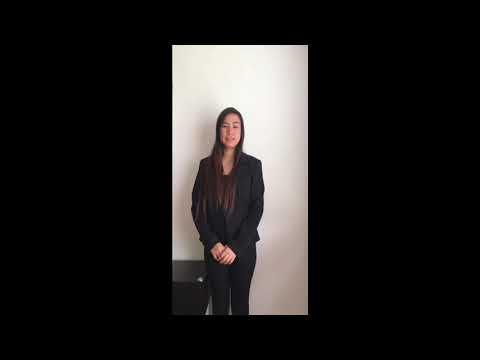The image depicts an Asian woman in a professional black suit, standing in front of a white wall. She appears to be between her late teens and early 30s. She has long, straight brown hair with darker roots, which reaches down to around her elbows or waist. The woman, who has a slightly darker skin tone, stands with her hands crossed, eyes partially closed, and mouth slightly open, suggesting she might be in the midst of speaking or smiling. The photograph is framed with thick black borders on all sides, making the captured image appear quite small and emphasizing its vertical orientation. The picture is cropped at her knees, showing her full figure up to her head, with an additional portion of the white wall above her. The overall setting is simple, with a potential hint of a black tabletop in the lower part of the image, which might be part of a video interview setup or a casual recording environment, adding to the professional yet approachable ambiance.